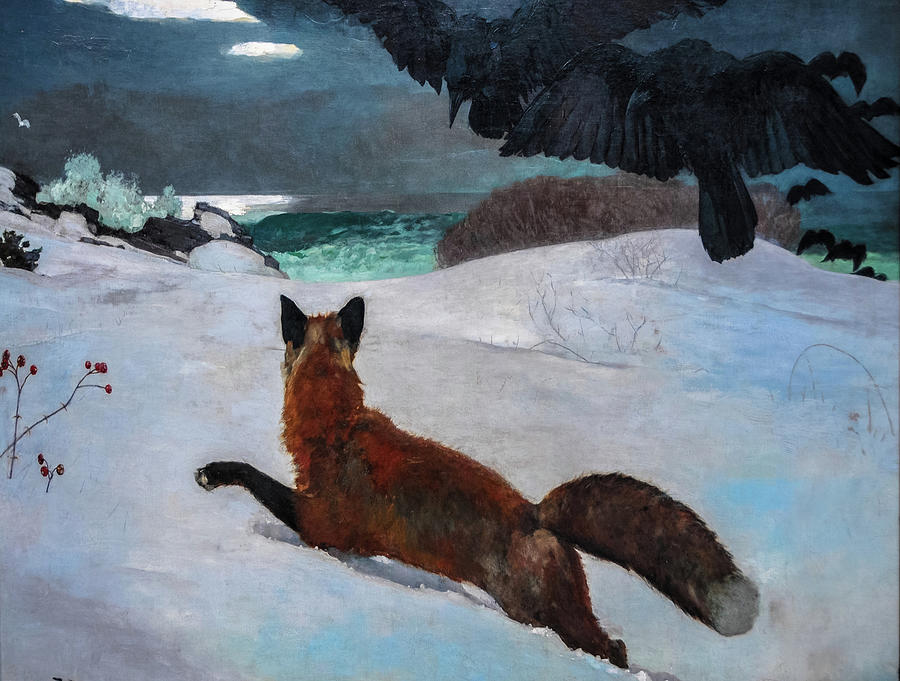This is a hand-painted image capturing a serene winter landscape featuring a red fox with a fluffy, brown-tipped tail running through deep, thick snow. The fox, characterized by its reddish-orange coat, brown ears, and brown paws, is depicted with its left front leg lifted, glancing into the distance. The snow appears fresh and untouched, with sparse thin stems and shrubs poking through the blanket of white. In the upper right corner, a hawk with widespread wings seems to be swooping down, adding a dynamic element to the tranquil scene. The background is peppered with hints of blue, turquoise, and green, suggesting the presence of a pond or the edge of an ocean, possibly reflecting the sky or moon, creating a natural gradient from the snow to the distant horizon. Also visible are dark, rocky forms that could be either rocks or penguins. This picturesque painting, set against a backdrop of distant mountains and snow-capped peaks, evokes a sense of peace and the wild beauty of nature.